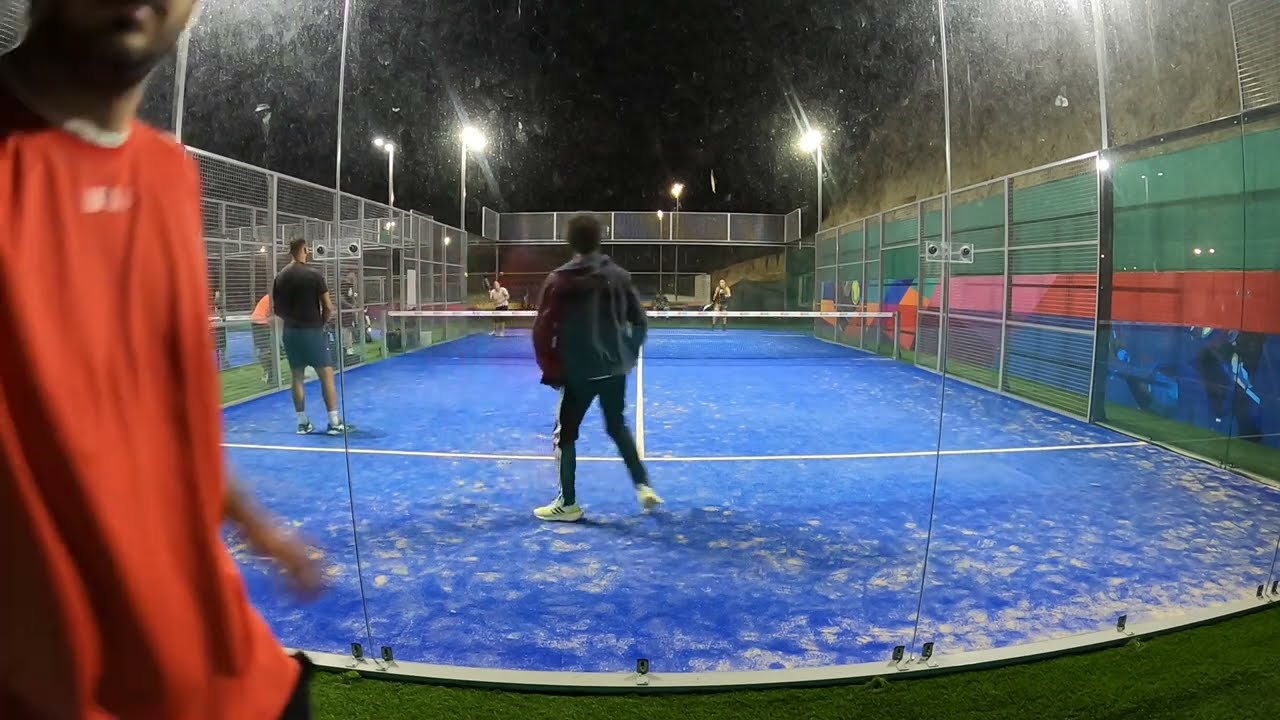The image depicts a nighttime tennis match on an outdoor tennis court with distinctive features. The blue court is worn in several spots, revealing underlying white patches that almost resemble snow. Surrounding the court is a chain link fence adorned with colorful paneling in shades of green, red, blue, and pink, contributing to the privacy of the setting. Additionally, one wall near the front is uniquely constructed from various acrylic panels held together by metal fasteners. The court's edges are lined with a dark green faux grass carpet.

The scene includes four men actively engaged in the game. One man on the left side is dressed in an orange shirt with a white collar and black pants. To his right, another player is captured in motion, wearing a long-sleeve gray jacket and long pants, with his right foot poised as if preparing to move. Slightly forward, a third man in a black shirt and gray shorts is also in action. Two more players are faintly visible on the opposite side of the court, both wearing shorts. In the foreground, the image partially frames a man in a reddish-orange t-shirt with tan skin, displaying his chin, lips, and blurred left arm in motion.

Bright lights illuminate the court, contributing to the slight blur of the image and casting a stark contrast against the dark night sky.